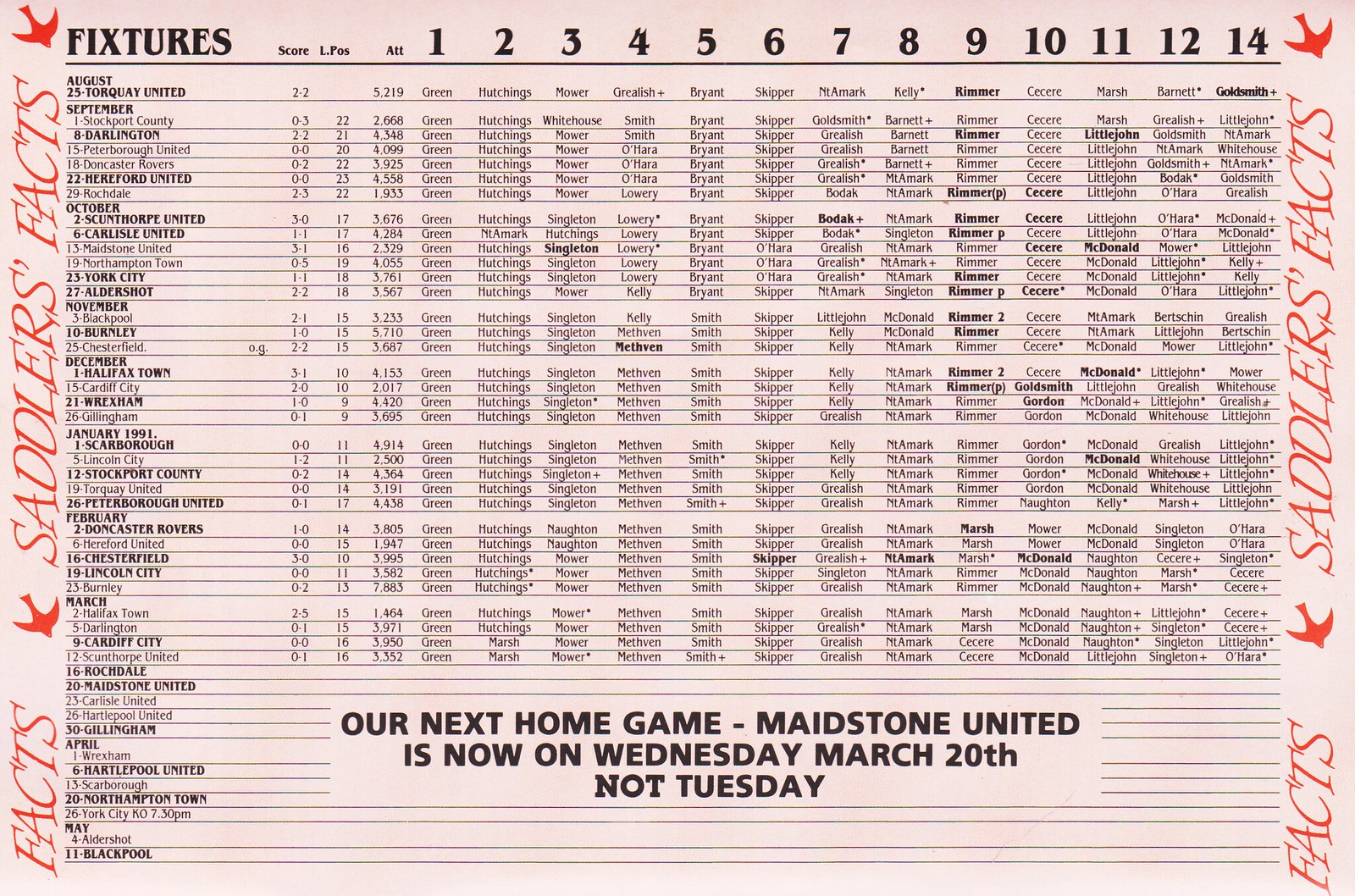The image is a horizontally oriented scan of a fact sheet or gameday magazine page, with a pinkish hue. Prominent red text on both the left and right sides of the page reads, "Facts, Sadler's Facts." The top left corner features multiple lines of black text, starting with column headers that read, "Fixtures," "Score," "L," followed by positions 1 through 12 and 14, notably skipping 13. The table lists dates and team names such as Torquay United, Hereford United, Darlington, and York City, with associated scores and other data. Running vertically along the right side are the words "Facts, Sadler's Facts." At the bottom, bold text announces that the next home game, Maidstone United, has been rescheduled to Wednesday, March 20th, instead of Tuesday.